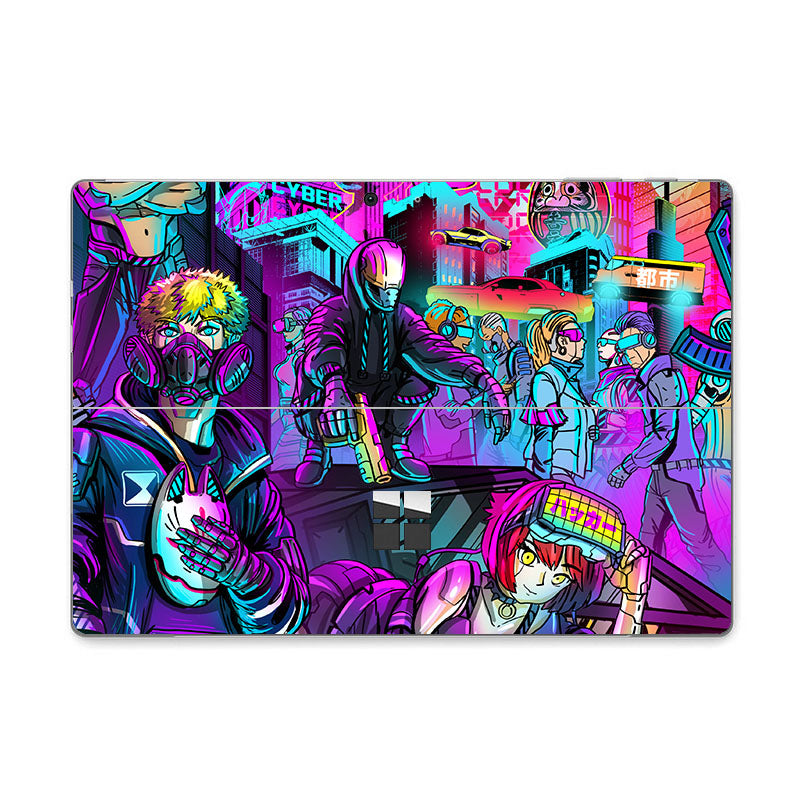This detailed, dystopian, cyberpunk-themed image is bathed in shades of purple and teal, incorporating a variety of figures and objects that contribute to its busy and chaotic scene. In the foreground, towards the bottom right, is a striking cartoon character with bright red hair, a choker, and a visor pulled up over her eyes, making her a prominent feature. On the left is a person with short blonde hair and blue eyes, wearing a gas mask and a hoodie adorned with a cat image partially obscured by their hand. Central to the image is a figure crouching down, equipped with a helmet reflecting the surrounding purple hues, a long-sleeved jacket, gloves, and holding a gun—adding an ominous edge to the scene. Surrounding these main characters are various other figures and objects, including street signs, cars, and buildings, all meshed together in a dense urban tapestry. The word "cyber" is visible, hinting at the overarching theme of a futuristic cyber city where people exhibit cybernetic features or wear futuristic gear, and vehicles, including flying buses with Japanese lettering, navigate the busy airborne traffic. The entire scene combines multiple colors - purple, black, white, yellow, orange, mint green, various shades of blue, brown, red, and pink - creating a visually rich and complex mural-like composition.